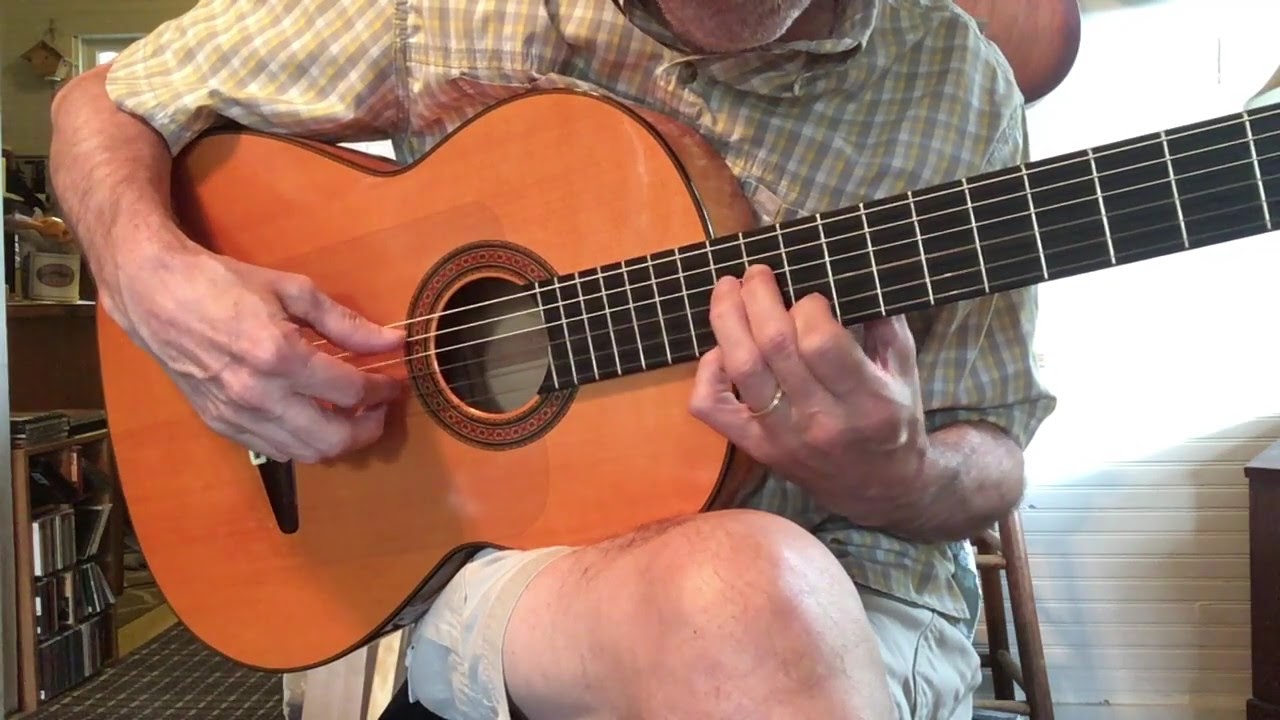The image captures a middle-aged man with grey stubble, indicating he is likely around 50 years old, sitting in a homey living room setting and playing an acoustic guitar with a polished wooden finish. He is adorned in a light green plaid shirt and jean shorts, and a gold wedding ring gleams on his left hand as he manipulates the chords. His posture is relaxed, with one leg crossed over the other, the guitar resting on the elevated leg. Although his face is predominantly obscured, his chin and jawline are visible. The background features a white brick wall and a bookcase filled with CDs, suggesting a music enthusiast’s sanctuary. To the left, shelves hold additional items including a jar and a quaint cuckoo clock in the upper corner, while a brown and white checkered rug covers the floor, adding to the room's cozy ambiance. The light source seems to emanate from behind, casting a soft glow over the serene scene.